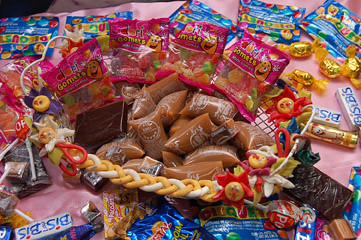The close-up image captures a festive gift basket centered on a table adorned with a pink tablecloth. Inside the basket, various types of packaged candies are arranged, including hard-to-identify sweets and prominently featured items like a big block of chocolate on the left and packages of caramel candies. The basket itself, possibly an Easter basket or for a similar celebration, has a whimsical design with little happy face suns or flowers. The centerpiece includes pink cellophane-wrapped assortments of multi-colored candies, likely hard candies and maybe sour gummies. Scattered around the basket on the table are an abundance of additional candy packages, predominantly blue, and several bars labeled 'bis bis'. Other noted sweets include butterscotch on the right-hand corner, lollipops in gold wrapping, and assorted fruity gummies, providing a delightful mix of treats ready for a celebration.